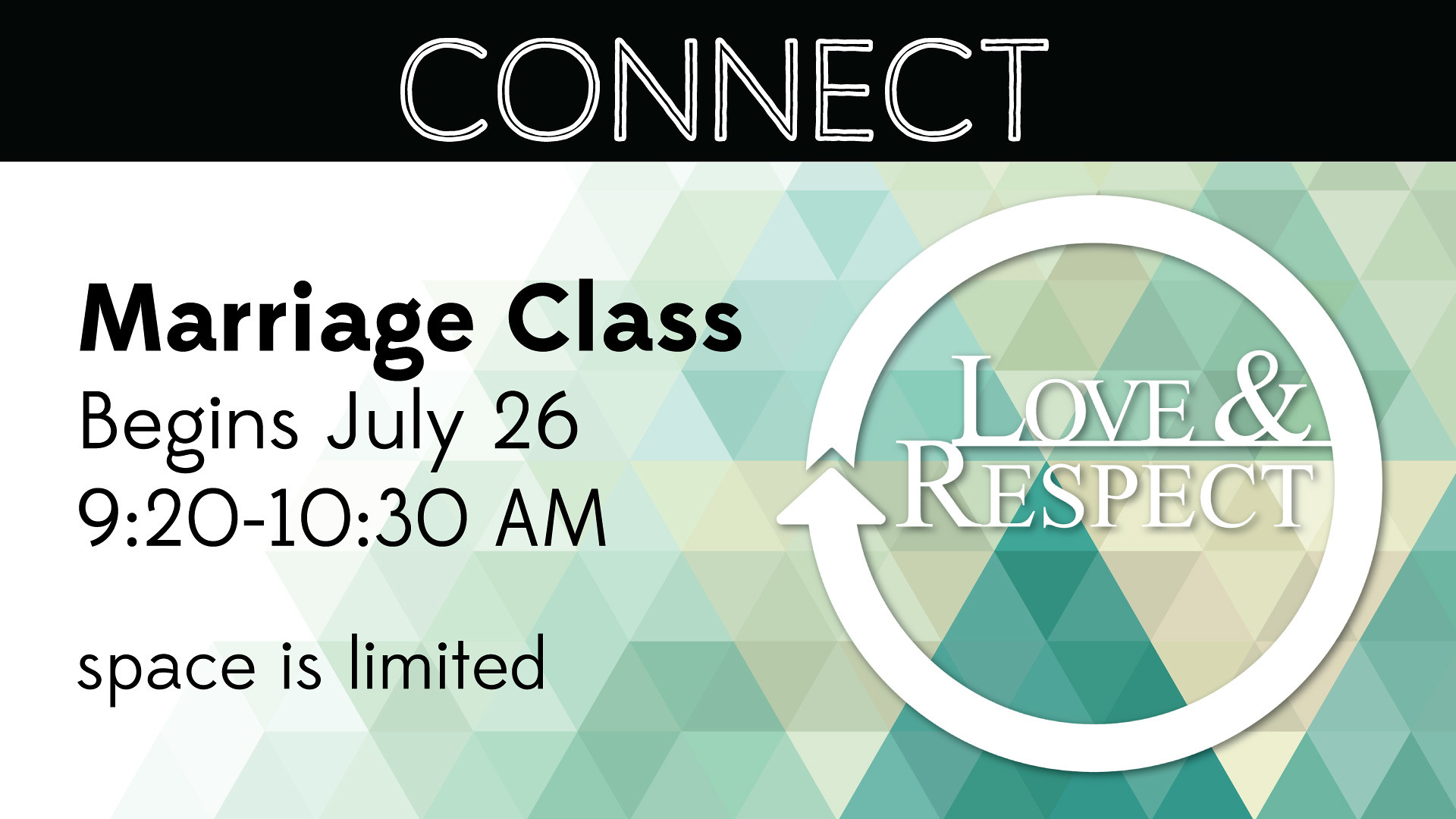The image is a digitally created advertisement set in a horizontal, rectangular format. At the top, a black, thin horizontal stripe spans the width of the banner, displaying the word "CONNECT" in bold, white capital letters. Below this, the background consists of a geometric pattern of green, olive, and off-white triangles that vary in size and shade, with lighter colors on the left transitioning to darker greens on the right.

On the left-hand side of the image, the text "MARRIAGE CLASS" is prominently displayed in bold, black letters. Beneath it, in a regular font, the text reads: "begins July 26th, 920-1030 a.m., spaces limited."

On the right-hand side, a white circle contains an arrow, which loops around, starting and ending within the circle, giving a sense of continuous motion. Inside the circle, the words "LOVE & RESPECT" are written in a clean, concise font. The background behind this circle features larger, darker green triangles, highlighting the graphic and creating a visual emphasis on the logo.

The coherent design and structured layout are unified by the geometric elements and the careful positioning of text, making it a clear and effective advertisement for the upcoming marriage class.